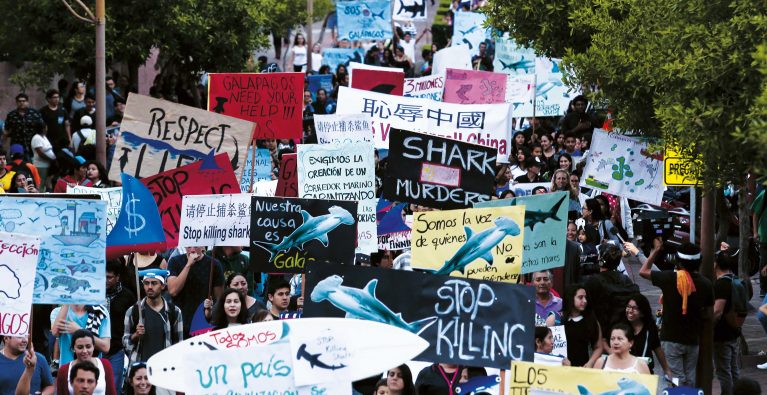The image depicts a vibrant daytime protest march on a tree-lined boulevard with wide sidewalks, filled with a throng of people advocating against the killing of sharks. The scene is buzzing with activists of various ethnicities, prominently Hispanic, Chinese, and others, holding an array of large, colorful signs. Some signs are emblazoned with intricate paintings of hammerhead sharks, while the messages are expressed in multiple languages including English, Spanish, Chinese, and French. Slogans such as "Stop Killing," "Nuestra Causa," "Somos la Voz," "Don't kill sharks," and "Galapagos needs your help" adorn the posters, highlighting the urgency and international concern over the issue, possibly related to practices like shark fin soup. The signs stand out against the diverse sea of protesters, showcasing an array of red, white, blue, tan, and pink backgrounds in this landscape-oriented color photograph.